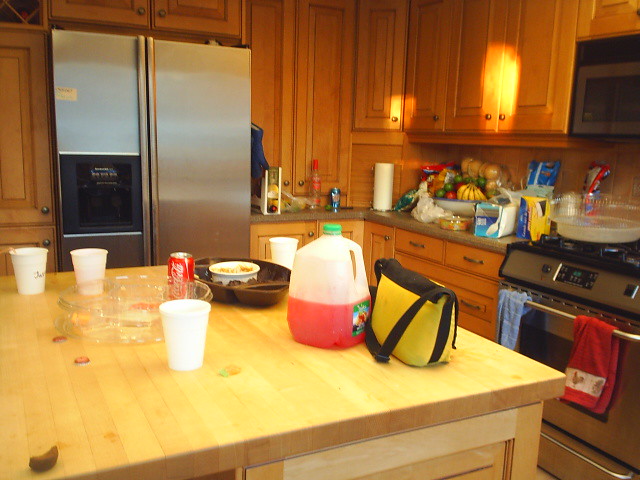A cozy kitchen featuring an array of wooden cabinets adorned with brass handles and knobs elegantly wraps around the room. Central to the space is a spacious wooden kitchen island, holding a five-liter bottle filled halfway with reddish-orange juice, capped with a green lid. Beside it, a yellow and black shoulder bag, a can of Coca-Cola, and three white plastic cups add to the scene's homely feel. Dominating one side, a large gas burner and substantial oven stand ready for culinary adventures, with a red and blue tea towel draped over the stainless steel handle of the oven doors. To complete the ensemble, a sleek double French door refrigerator with an ice dispenser stands prominently in the backdrop.